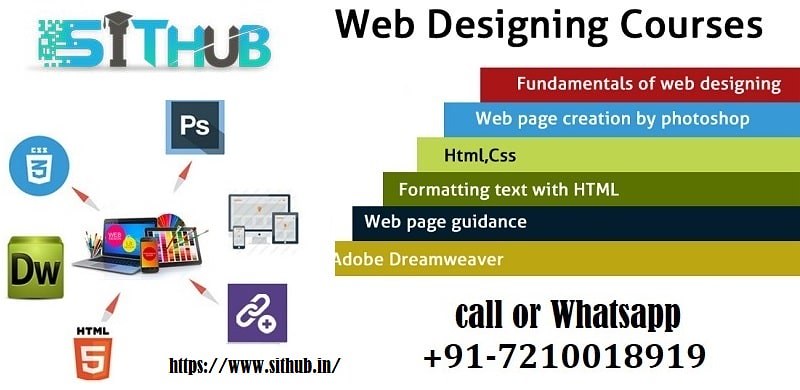The image is a chaotic infographic web advertisement for web designing courses. At the top left, there is a logo that spells out "Sithub," with a distinctive design where the "I" is a podium topped with a graduation cap, and the "U" is in black while the other letters are in light blue. Below the logo, there is a graphic featuring a laptop and a tablet with arrows pointing to various icons, including Photoshop, Dreamweaver, HTML5, CN, and a TV logo.

On the right-hand side, "Web Designing Courses" is prominently displayed in black font. Below this, there are six colored bars descending from the top right to the bottom left, each containing white text detailing different components of the courses. The bars are as follows:
1. Red bar: "Fundamentals of Web Designing"
2. Blue bar: "Webpage Creation by Photoshop"
3. Bright green bar: "HTML CSS"
4. Dark green bar: "Formatting Text with HTML"
5. Black bar: "Webpage Guidance"
6. Yellow bar: "Adobe Dreamweaver"

At the bottom right corner, it says "Call or WhatsApp +91-7210018919" in a clear format.